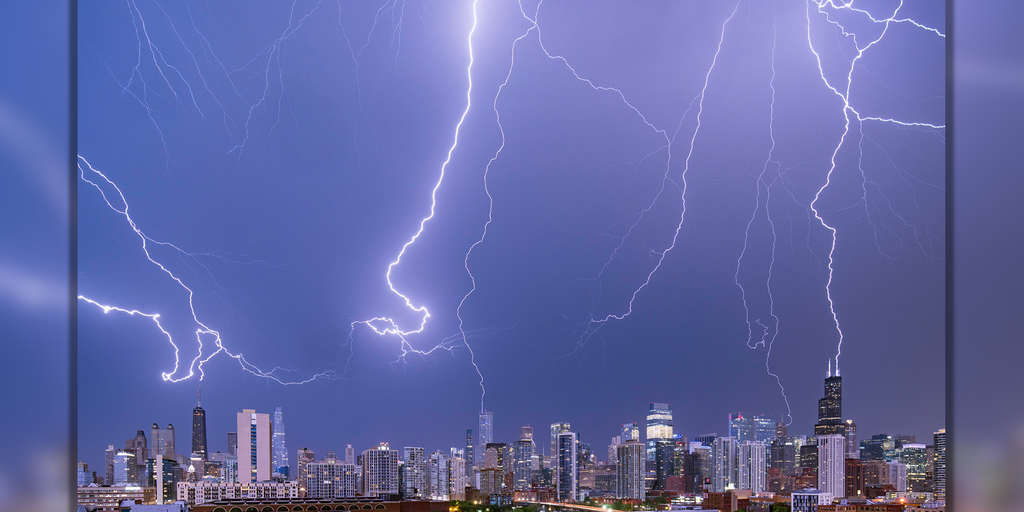A breathtaking photograph captures a vibrant cityscape during the evening hours, viewed through a clear glass window framed by two black window panes. The city's skyline stretches across the image from left to right, with numerous buildings illuminated, casting a warm and inviting glow. Above the city, a dramatic sky showcases multiple lightning strikes, each one delivering a shocking burst of energy to the urban landscape below. The lightning bolts, luminescent in neon hues of white and light blue, create an electrifying contrast against the darkening sky. A particularly striking bolt is seen making contact with a tall, black building situated in the upper right corner of the scene, emphasizing the raw power and beauty of nature as it intersects with the man-made environment.